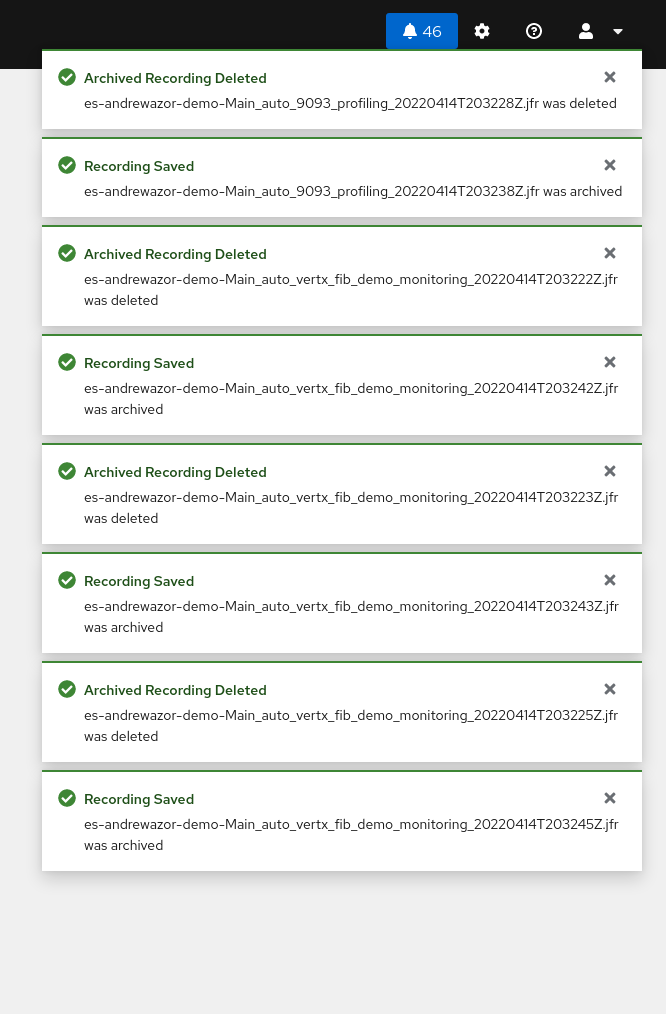The top section of the image features a black background with a blue circle containing a white bell icon and the number 46 beside it. To its right, there is a settings wheel icon. Below this header, a sequence of elongated horizontal rectangles is displayed. Each rectangle includes different elements.

In each rectangle:
- A green box with the text "Archived Recording Deleted" appears first.
- This is followed by a long web address consisting of a mix of letters and numbers.
- Next, there is another green box with a white checkmark inside and the text "Recording Saved."
- The rectangles contain these elements multiple times, consistently alternating between "Archived Recording Deleted" and "Recording Saved" messages.

Each rectangle also has a clickable 'X' on the right side, allowing users to remove the information. There are eight such rectangles in the center of the image. 

The overall structure consists of repetitive patterns of green notification boxes indicating the deletion and saving of recordings, punctuated by web addresses and an 'X' for easy removal, all situated beneath the initial header.